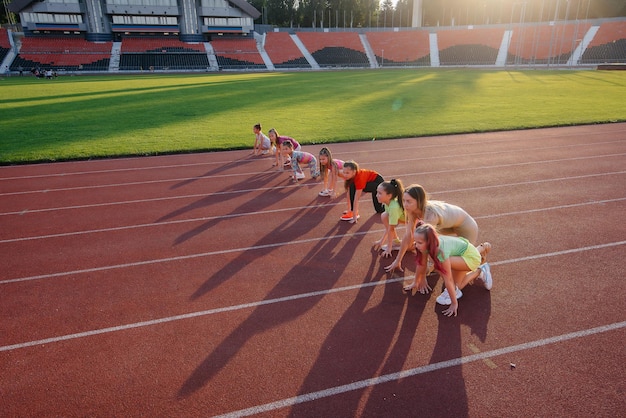This photo captures an outdoor track and field event at an empty stadium. A group of young girls, each in their own lane, are lined up on a reddish-brown, clay-colored track, marked with white lines. They are in starting positions, facing left, with the sun casting their shadows diagonally across the track in front of them. Each girl is wearing athletic outfits, ready to begin the footrace. The surroundings include well-maintained green grass next to the track, and in the background, there is an expanse of stadium seating that is orange at the top and black at the bottom. Trees and a green field further frame the scene, with an enclosed announcer area positioned on the far left. The image is serene and captures the anticipation of the moment just before the race starts, with the empty audience seats emphasizing the focus on the athletes and their upcoming competition.